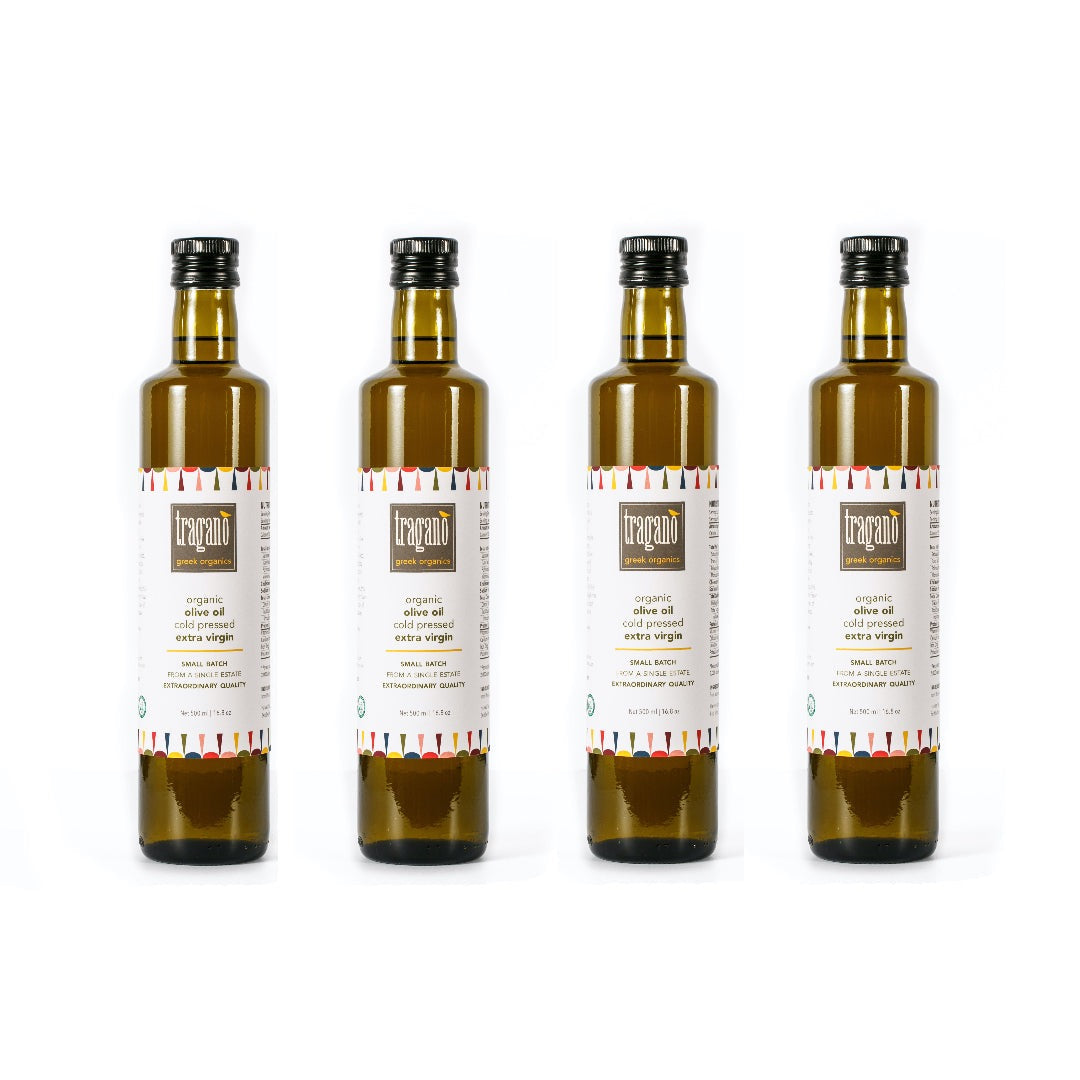In this image, we see four tall, slender bottles of organic, cold-pressed, extra virgin olive oil, arranged side-by-side against a completely white background. These are premium, small-batch oils of extraordinary quality, likely sourced from Greece, given the text on the labels. Each bottle appears to be made of a light brown, see-through material that resembles glass or potentially plastic. 

The labels, which cover a significant portion of the bottle's height, are predominantly white with a central brown square near the top. In this square, "TRIGONO" is inscribed in white text, with a charming yellow bird perched on the final "O." Beneath that, the words "GREEK ORGANICS" are printed in orange. Further down, the label sequentially features the words "ORGANIC," "OLIVE OIL," "COLD PRESSED," and "EXTRA VIRGIN" in clear, organized text. The oil inside these bottles has a yellowish hue, indicative of high-quality olive oil, and each bottle is capped with a solid black top. The overall presentation exudes a sense of elegance and premium quality.